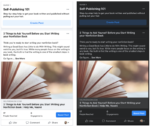This image showcases a user interface presented in two modes: light mode and dark mode. The interface is split into two side-by-side pictures for comparison. On the left side, the background is white with black text, representing light mode. On the right side, the background is black with white text, depicting dark mode. Both sides feature a light blue button with dark blue text at the top and another blue button with white text at the bottom right. Centrally located near the bottom of both images is a brown graphic element. The overall text in both versions is small and blurry, making it difficult to read, but the color contrast between the text and backgrounds is clearly visible.